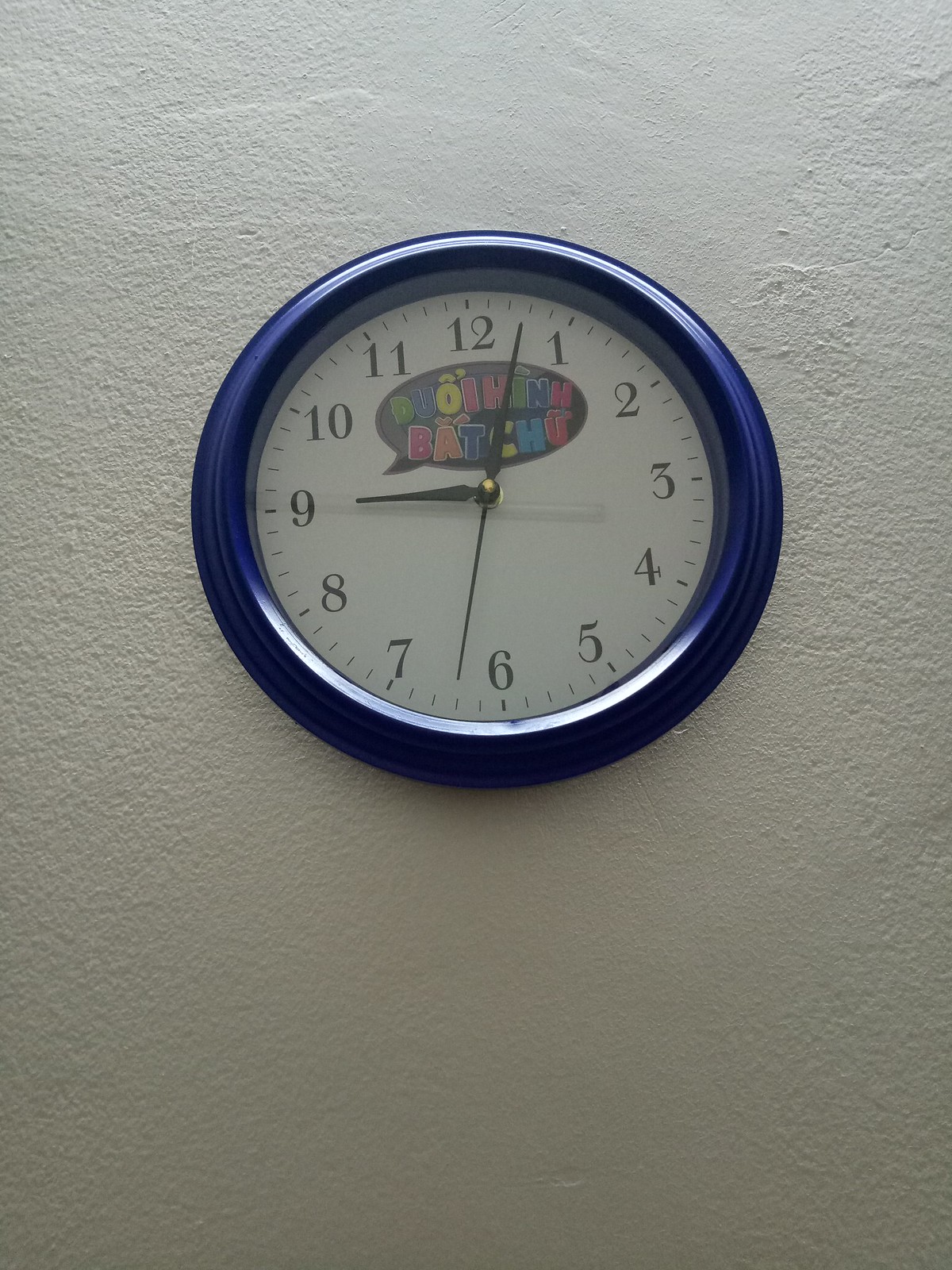The photograph features a clock positioned slightly above the center. This clock boasts a thick blue rim that frames its white face. Along the outer edge of the white face, there are fine straight lines indicating the minutes, with bolder, thicker lines marking the hours. The numbers, rendered in black, are clearly visible against the clean white background. At the heart of the clock, a gold circle anchors the hands, which are all black including the second hand. Below the number 12, an oval shape extends nearly to the numbers 10 and 2. This black oval contains colored letters, though they are unreadable in the picture. The clock displays the time as 9:03.